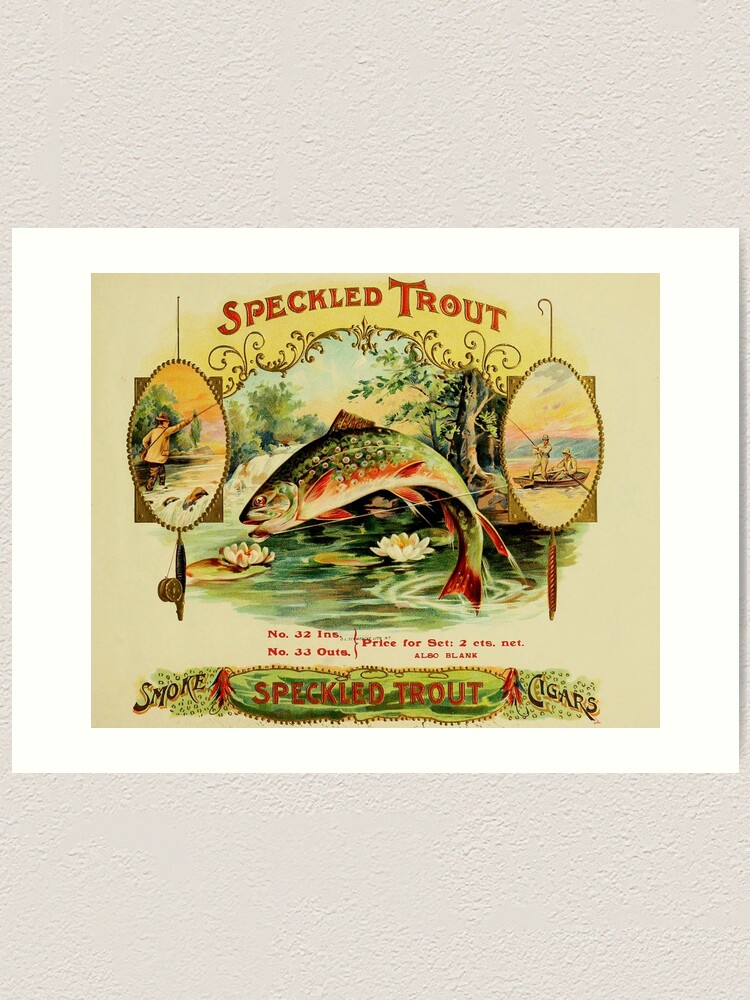The image is a vintage advertisement poster for "Speckled Trout Cigars," with the main background displaying a light beige or grayish hue, bordered by white at the top and sides. The poster prominently features the words "Speckled Trout" in ornate, reddish lettering at both the top and the bottom, the latter set against a green backdrop and accompanied by "Smoke Speckled Trout Cigars." An illustration at the center depicts a trout leaping from a serene, lily-dotted pond, backed by a peaceful sky and tree-studded horizon. Flanking the trout, there are two oval vignettes: one showing a fisherman standing in a stream, and the other depicting two anglers in a boat. Additional text details the price of the cigars, noting "number 33 ins, number 33 outs, price per set, 2 cents net." The scene is rich in color, further enhancing the classic, nostalgic feel of the advertisement.